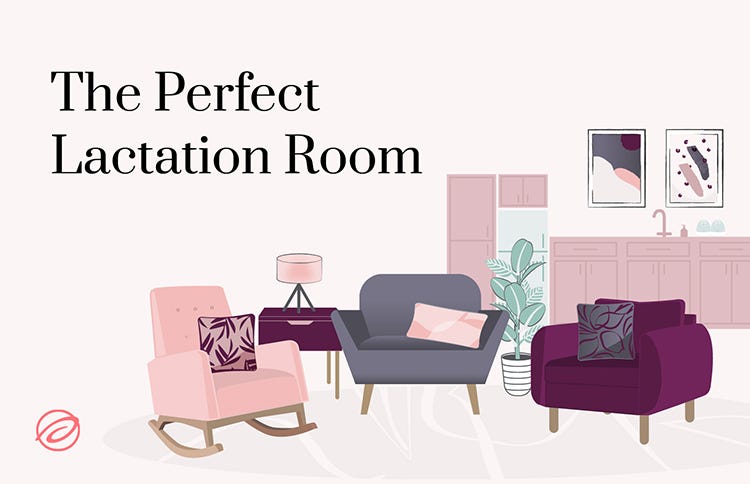This image is an animated graphic titled "The Perfect Lactation Room" in bold black lettering located in the upper left corner. The background is a subtle, nearly imperceptible blush-pink hue. The foreground presents a cozy room setup featuring three distinct chairs: a magenta easy chair with a matching magenta and gray pillow, a gray easy chair with a pink pillow, and a light pink rocking chair adorned with a pink and magenta pillow bearing fern illustrations. 

A side table accompanies the chairs, topped with a magenta lamp that has a pink lampshade. Adding a touch of greenery to the room, a white plant pot with a flourishing green plant is positioned behind the seating area. 

In the background, there's a kitchen section with pink cabinetry and a white fridge with a greenish tint. This area is decorated with abstract paintings that incorporate a palette of whites, pinks, grays, and magentas. Finally, a logo resembling a pinkish-reddish circle with a wave-like swirl can be found in the bottom left corner of the image. The entire scene is designed to exude a serene and welcoming atmosphere, ideal for a lactation room.